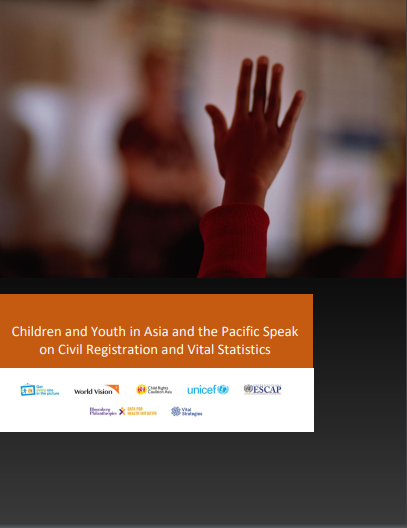In the foreground of the image, a child's right hand is prominently raised, as if participating or asking a question. The hand, adorned with thin fingers and tan skin, belongs to someone wearing a long, red, long-sleeve shirt. The background features a blurred classroom setting. To the left, there's a woman in a black outfit with crossed arms, observing the scene with a slight curve to her posture. A whiteboard is partially visible behind her, adding to the educational environment.

Beneath this main scene, in the lower center, there's a white and orange box. The orange section at the top contains white text that reads, "Children and youth in Asia and the Pacific speak on civil registration and vital statistics." The white section below it features various organizational logos, with "World Vision" in black text, "UNICEF" in blue text, and "ESCAP" in dark blue text among them. Smaller logos are also present, though they are hard to decipher. This white and orange box is set against a darker gray box, which serves as a subtle background element.